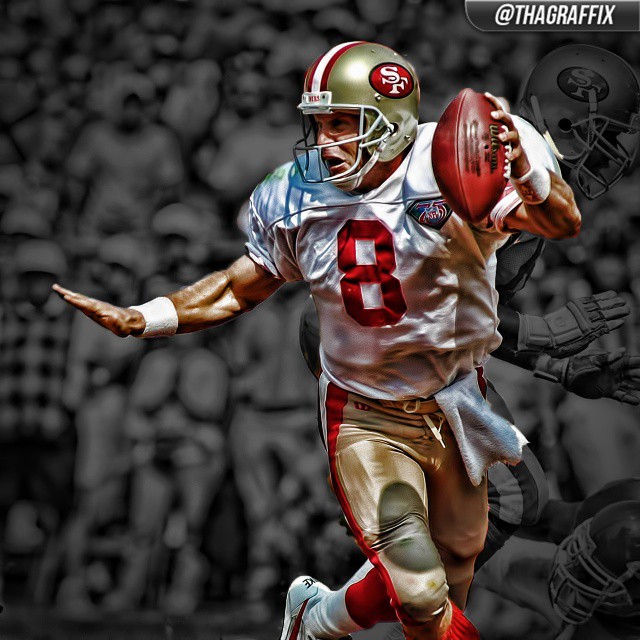This is an action-packed photograph or football card featuring NFL player Steve Young. In the image, Young is captured mid-run, dashing towards the right side of the frame. He is holding a football securely in his left hand while extending his right arm out to the left, possibly for balance or to block an incoming opponent. His intense focus is evident as he looks to the left with his mouth slightly open, perhaps catching his breath. Young is donning the iconic white jersey with a striking red number 8 of the San Francisco 49ers, complemented by white shoes and a distinctive gold helmet with red and blue details. The dynamic scene is set against a superimposed black and white background which features an image of Young, and possibly a crowd, adding depth and a sense of motion to the card. The top right corner of the card displays the text "AT-THA-GRAPHICS" in white. Overall, this detailed and layered composition not only captures Young in action but also emphasizes his prominence on the field.